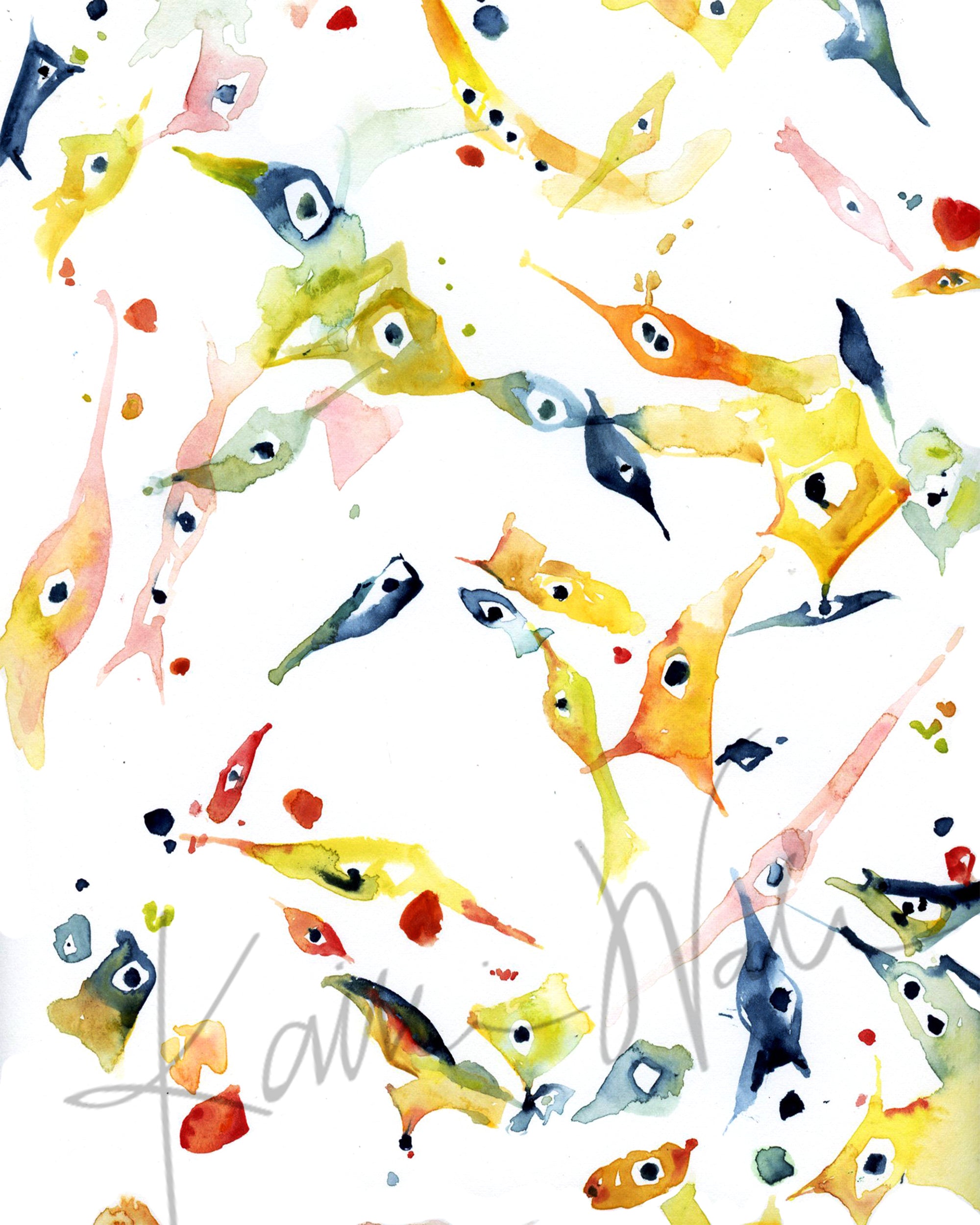This watercolor painting, set against a stark white background, depicts an array of vibrant, multi-colored entities resembling fish or single-celled organisms. Each figure, bursting with hues of green, yellow, blue, pink, red, orange, and teal, features a singular eye with a central black spot, adding a curious life-like quality. The spontaneous brushstrokes give the impression that the paint was briskly thrown at the canvas, resulting in dynamic streaks and splashes of color. Scattered across the canvas, these figures number between 20 to 30, and their lively colors contrast sharply with the smooth white backdrop. At the bottom, in gray cursive lettering, is what appears to be the artist's name, "K-A-W-U-O-N-W-A-U-O-L-I," hinting at the creator's identity.